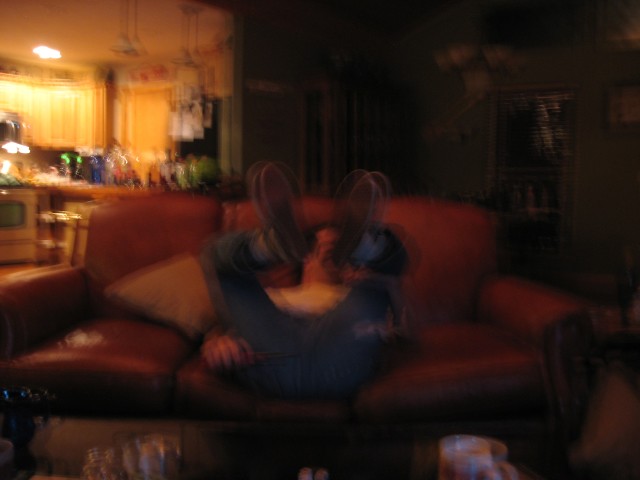The photograph, taken indoors, is a blurry and poorly lit color image capturing a scene at night in what appears to be someone's apartment or house. At the center of the image, a man is reclined on a red, three-cushion sofa that dominates the living area and seamlessly transitions into a visible kitchen in the background. The man, dressed in a white t-shirt and fitted blue jeans with legs bent at the knee, has his feet pointing upward and his right hand holding what looks like a lighter towards his rear end, suggesting a comedic intent to light something expelled. His dark hair is barely visible as his head is obscured by his shoe, making his face indistinguishable. Illumination comes from a single kitchen light that casts a faint glow over wooden-finished cabinets and a cluttered countertop populated with bottles. The foreground features what appears to be a black coffee table with miscellaneous items, including a coffee cup, partially in frame. The right side of the image remains shrouded in darkness but hints at additional furnishings like a window, door, and chandelier.